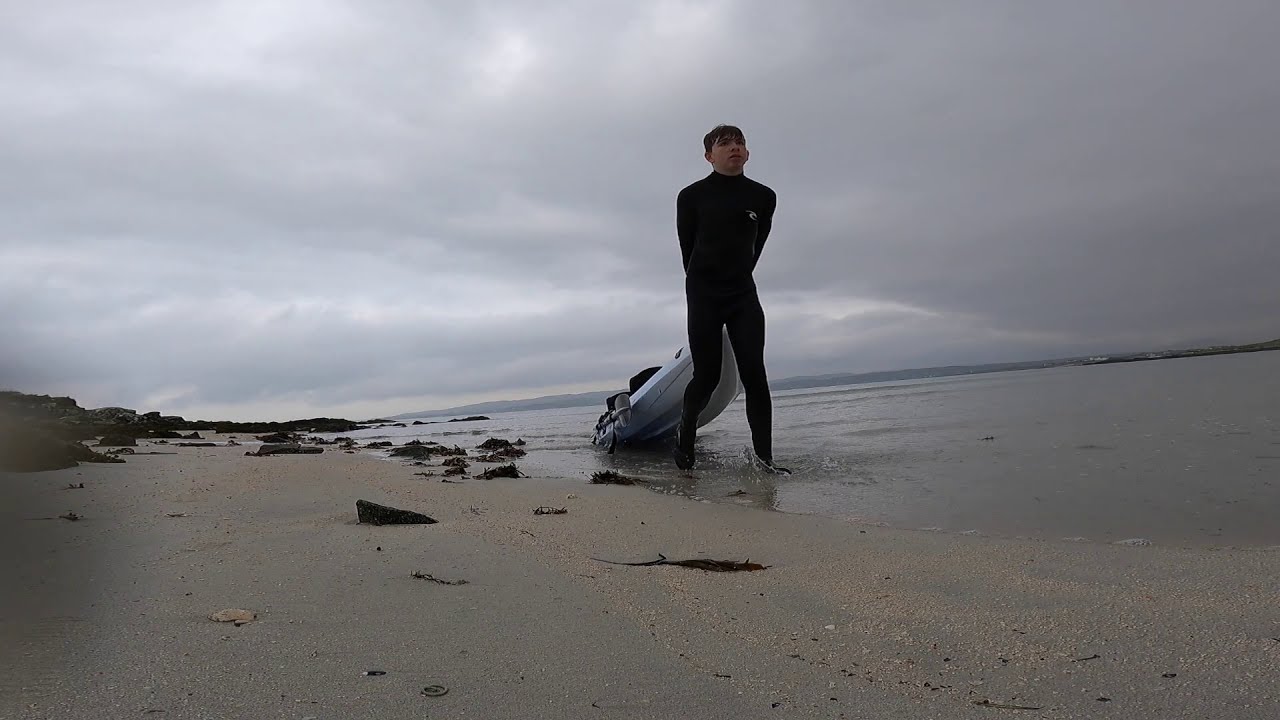This high-definition photograph, captured during a dreary winter day, portrays a stark yet serene beach scene. Dominating the center of the image is a young man, perhaps in his twenties or thirties, with wet black hair laying flat on his head. Clad in a black, full-body wetsuit, he strides across a sandy, rocky beach, towing a white kayak—or possibly a very thin canoe—behind him. The water appears on the right side of the image, while the sandy shore extends from the lower right-hand corner towards the center-left. The backdrop is a tumultuous sky, heavy with dark gray clouds that suggest an impending storm, further emphasizing the desolate ambiance. Despite the somber setting, the young man's muscular build and purposeful movement add a dynamic element to the scene. White light pierces through the clouds, juxtaposing against the darker hues and illuminating the shoreline where he treads. The overall composition, with its elements of water, sand, and foreboding sky, evokes a powerful sense of solitude amidst nature's vastness.